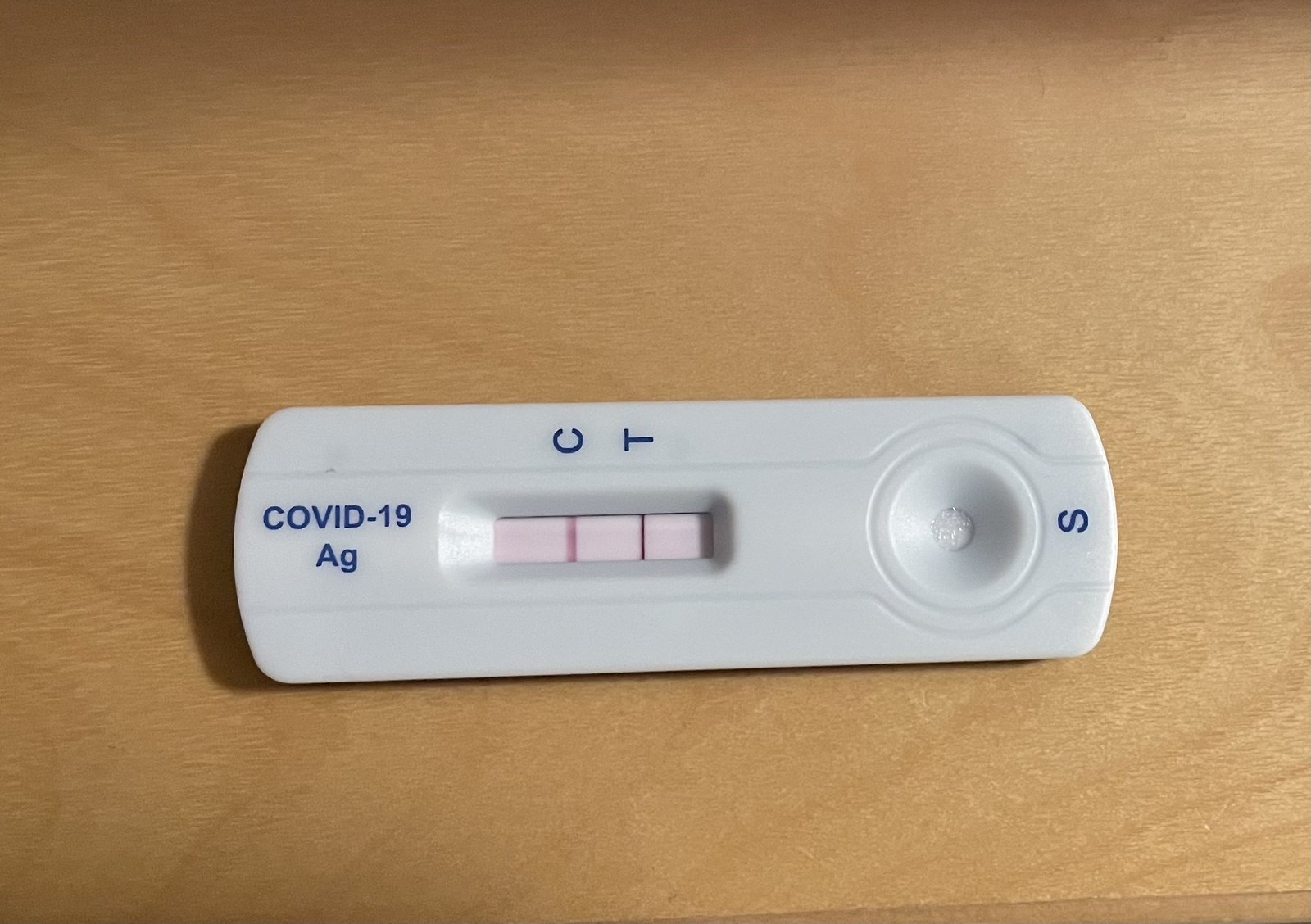A horizontally positioned COVID-19 antigen test lies flat on a smooth, light-colored wooden table. The white rectangular test, distinguished by its curved edges, prominently displays "COVID-19 AG" on its surface. In the results window, marked with 'C' and 'T', two purple lines are visible: the 'C' line is slightly wider and less solid, while the 'T' line is thinner but distinct. At the bottom of the test, an 'S' indicates the sample area where the liquid is applied. The wooden table beneath is clean and devoid of any dust or specks, further emphasizing its smooth texture.